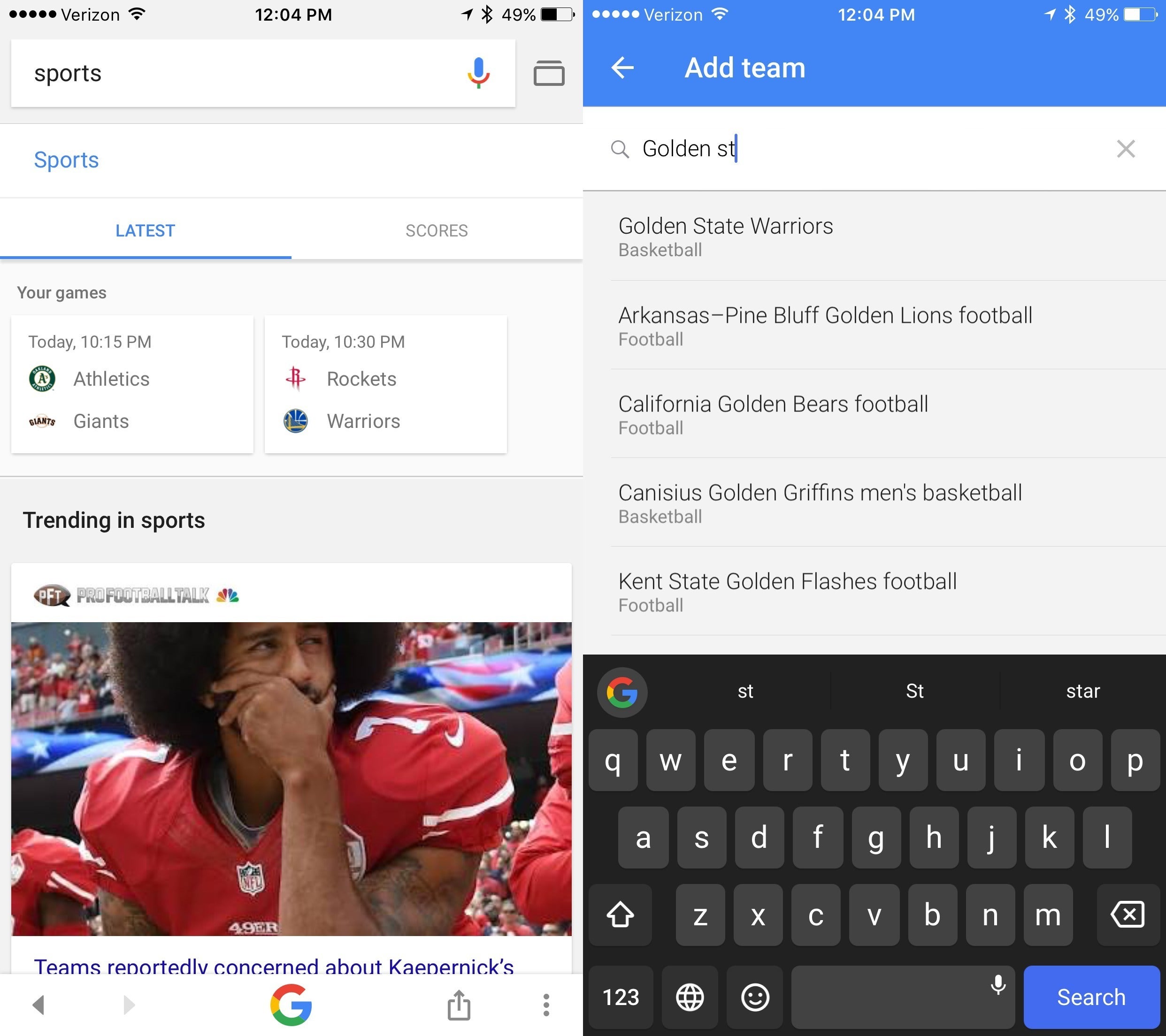The image is split into two parts, each displaying different information from a smartphone interface. 

**Left Side of the Image:**
- The top section features a light grey background with a search bar labeled "Sports." 
- A colorful Google microphone icon, in shades of blue, red, green, and yellow, is included within the search bar.
- Below the search bar, there are two tabs: "Latest" and "Score," with the "Latest" tab highlighted.
- The "Latest" tab shows the latest sports games and results under the heading "Your Games":
  - "Today, 10:15 PM - Athletics vs. Giants"
  - "Today, 10:30 PM - Rockets vs. Warriors."
- Further down, under the heading "Trending in Sports," there is an image of a football player wearing a red Nike jersey. The partially visible headline reads: "Team reportedly concerned about Keith Hendricks," with remaining text obscured. The headline text is in purple.
- At the bottom, the colorful Google logo, represented as a G with red, yellow, green, and blue segments, is displayed.

**Right Side of the Image:**
- The top of the screen displays various status icons, including a badge indicating 49% battery life, Bluetooth, the current time (12:04), signal strength, Wi-Fi, and the service provider, Verizon.
- Below this, a header with a blue background reads "Add Team."
- Beneath the header is a search box containing the text "Golden ST."
- There are additional search suggestions related to sports teams listed below: 
  - "Golden State Warriors (basketball team)"
  - "Arkansas Pine Bluff Golden Lions football team"
  - "California Golden Bears football"
  - "Kansas Golden Griffins men's basketball"
  - "Kent State Golden Flashes football."
- At the bottom of the screen, a black keyboard with white letters is visible, featuring a blue search button on the bottom right.

This comprehensive view highlights various sports-related search features and real-time data accessible via a smartphone interface.